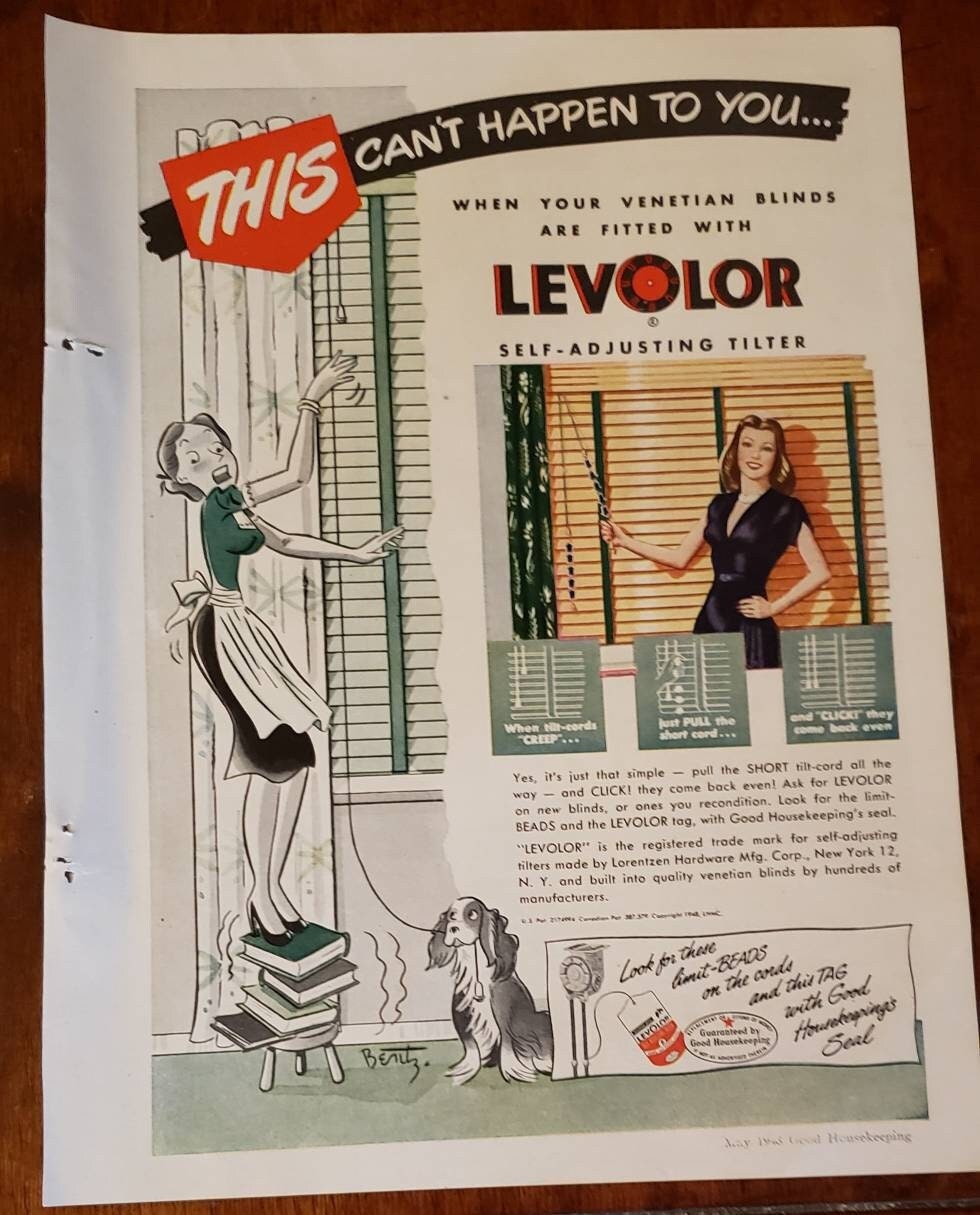The image depicts a vintage magazine advertisement for Levolor self-adjusting Venetian blinds. At the top, the ad features bold white text on a red, upside-down pentagon that reads, "THIS CAN'T HAPPEN TO YOU...". Beneath this, it continues with, "When your Venetian blinds are fitted with Levolor self-adjusting tilters". The center of the ad showcases a woman with long blonde hair wearing a black dress; she is holding a control pulley for the blinds with her right hand while her left hand rests on her hip. The background includes illustrations detailing the product's benefits: one cartoon depicts a maid precariously balanced on a stack of books, struggling to reach the blind adjuster, with a dog pulling on the other end of the cord. Additional text emphasizes the ease of use and reliability of Levolor blinds, highlighting the features such as limit beads and the Good Housekeeping Seal. The ad concludes with details about Levolor being a registered trademark of Lorenzen Hardware Manufacturing Corp, with a recommendation to ask for Levolor on new blinds or when reconditioning existing ones. The entire advertisement is printed on a piece of white paper placed on a brown wooden platform.